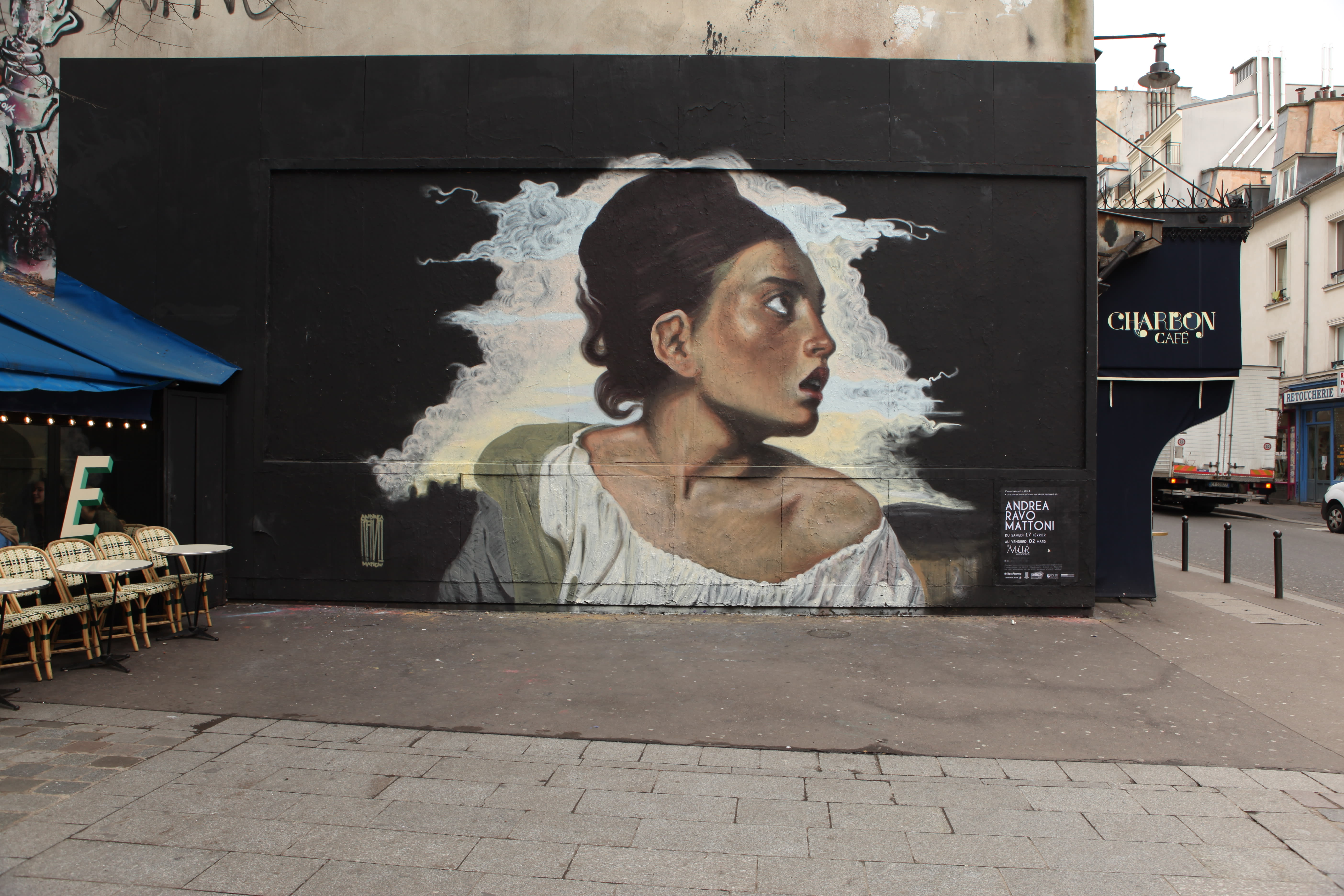This photograph captures the exterior of a building, possibly in Europe, adorned with a detailed mural. The background of the mural is jet black, covering the stucco wall, with a smoky white and gray area in the center framing the artwork. Prominently featured is the profile of a woman with olive skin and brown hair styled in a large bun, with some hair draping down her neck. She appears to be looking left, over her exposed left shoulder, which is bare due to her white peasant blouse slipping off. Her right shoulder is partially covered by an olive green jacket, nearly falling off. The woman's expression is one of alarm, and she has notable shading around her eyes and what appears to be a bruise on her right cheekbone. Below the mural, the artist's name, Andrea Ravo Mattoni, is inscribed. The building, which is likely part of an outdoor café, features "Charbonne Cafe" in yellow text on a sign facing the street and "Charbon Cafe" in white on a canvas awning. The scene includes an outdoor dining area with chairs and umbrellas on a beige cobblestone or tiled pavement, situated on a narrow street with cars and other buildings visible in the background.